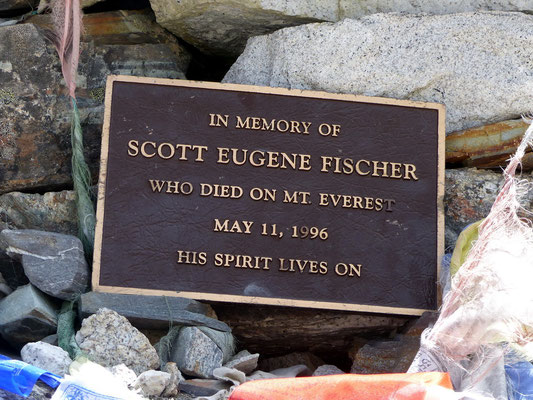The image depicts a rectangular plaque resting atop a collection of rocks and stones. The plaque is prominently centered in the image, crafted with a brown base, a gold-colored border, and gold lettering that reads, "In memory of Scott Eugene Fisher, who died on Mount Everest, May 11th, 1996. His spirit lives on." This tribute appears weathered and worn, suggesting it has been in place for a considerable time. Surrounding the plaque are various stones, including a large white stone speckled with black on the right and a chipped brown and white stone on the left. The background features boulders, one of which is dark gray while another is white with tiny black speckles. Among the rocks in the lower corners of the image, there are some unidentified objects—a blue item on the left and an orange item on the right. Additionally, a frayed rope, pink and transitioning to green, can be seen along with the presence of what might be cotton or cobwebs in the lower right corner.